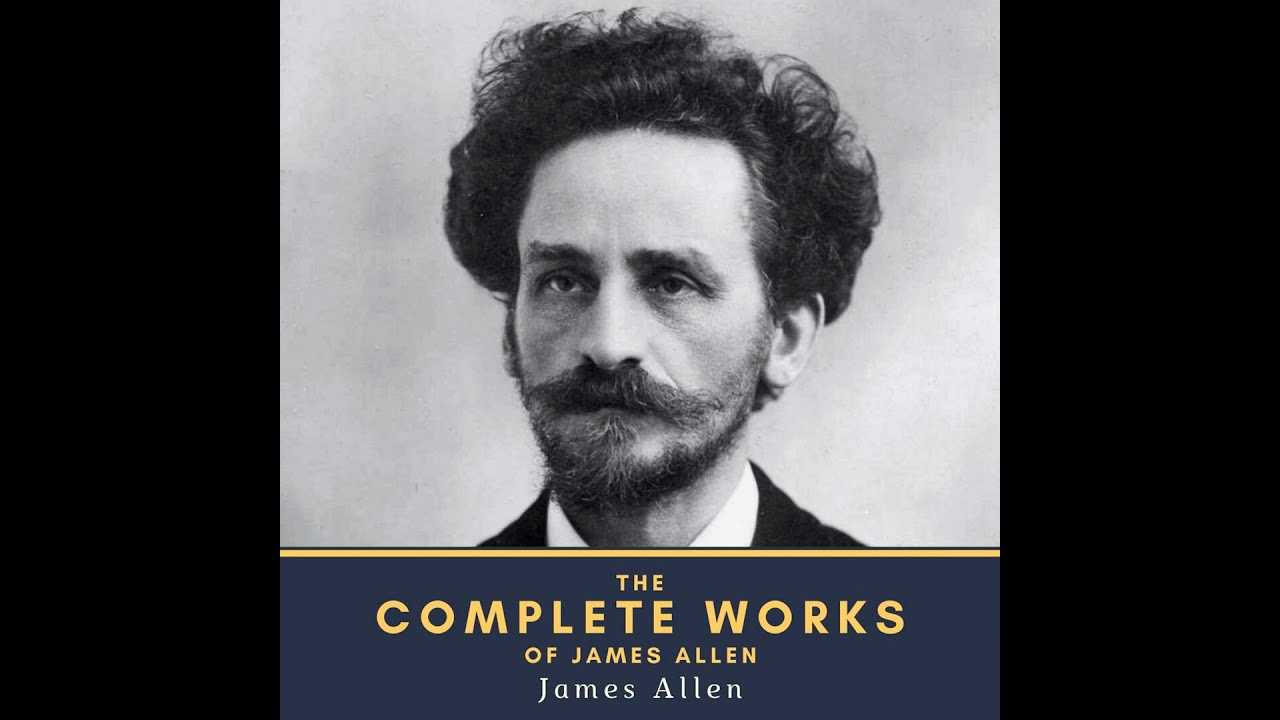This image is the cover of a book, featuring a black-and-white photograph of a man identified as James Allen. He appears to be a white male with thick, dark, and frizzy hair that is slightly messy and curls at the edges. His facial hair consists of a thick mustache that curls up at the ends and a goatee, complemented by really thick eyebrows. He is dressed in a black suit with a white shirt collar visible underneath. The man's expression is serious with a somewhat sad demeanor. The background of the cover is a dusty gray color. 

Above his photo, the top of the cover is black, while the middle part prominently displays the black-and-white photo of James Allen. Below his photo, there is a navy blue rectangle with a gold stripe running across it. In bold, large yellow letters, it reads "THE COMPLETE WORKS OF JAMES ALLEN," with "Complete Works" being the largest text on the cover. Directly beneath this text, in smaller white letters, is the name "James Allen."